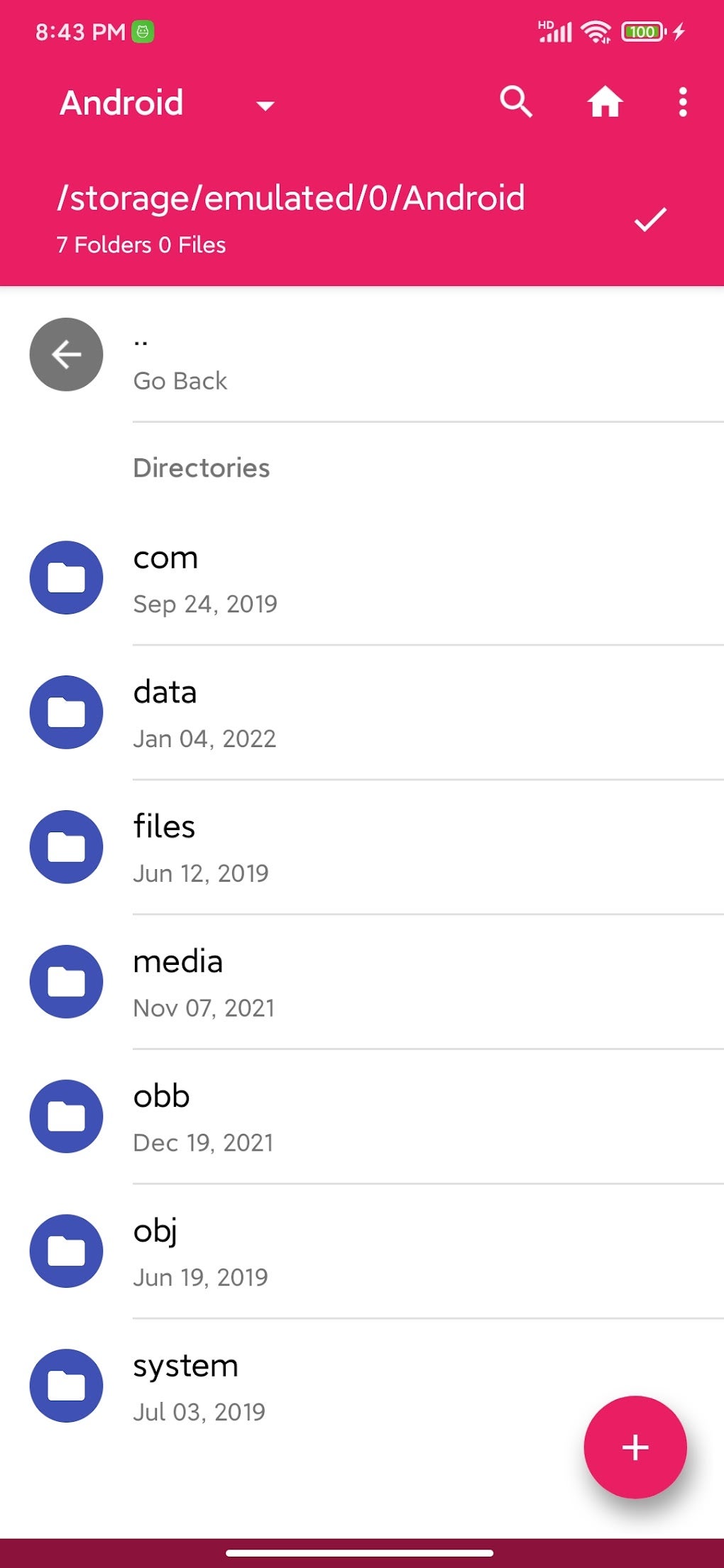This screenshot captures the user interface of a file management app on an Android cellphone. At the top, a bright pink header displays the time "8:43 PM" in white text on the left. Below this, the word "Android" is written beside a downward-pointing white arrow. On the right side of the header are three icons: a white magnifying glass for search functionality, a white house icon for the home screen, and three vertically-stacked white dots indicating additional options.

Directly beneath the header, the current directory path "/storage/emulated/0/Android" is shown in white text. To the right, a white check mark is present, followed by a small white text indicating, "7 folders, 0 files."

The main content area has a white background segmented by thin light gray lines, dividing several items. The first segment features a gray circle with a left-pointing white arrow next to the text ".." with "Go back" beneath it. This area is labeled "directories."

The following list includes:
- "com" with a date of "September 24, 2019," illustrated with a blue circle containing a white folder icon.
- "data" dated "January 04, 2022"
- "files" dated "June 12, 2019"
- "media" dated "November 7, 2021"
- "OBB" dated "December 19, 2021"
- "OBJ" dated "June 19, 2019"
- "system" dated "July 03, 2019"

In the bottom right corner, there is a floating pink action button with a white plus symbol, casting a medium gray shadow.

This detailed caption provides a comprehensive description of the file management app's interface, highlighting both visual and textual information.